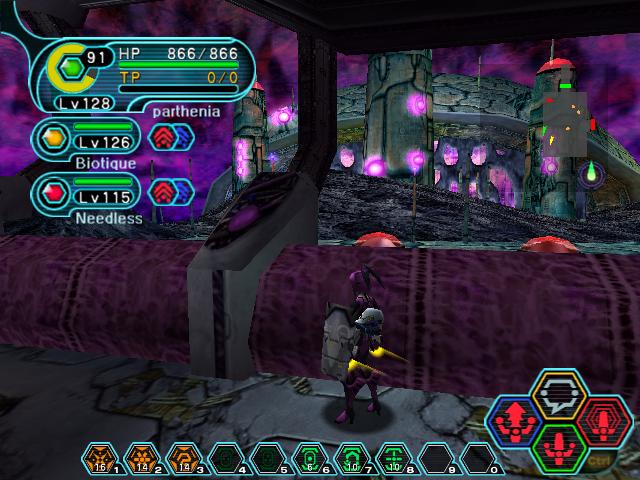A screenshot from a video game is depicted in this rectangular image. The scene presumably originates from a role-playing game, although the specific title remains unidentified. The environment showcases a diverse palette dominated by gray, burgundy, red, and pink hues, with occasional pops of green. Despite the unclear specifics of the setting, it appears to be an exterior location.

Centrally featured is a character who seems to be armed with guns, though the details are somewhat blurred. The character's health is indicated as HP 86/86. Above the character, labels such as "Parthenia," "Biotech," and "Needless" are visible, likely denoting various in-game elements or abilities.

The bottom segment of the screen displays additional information, possibly related to the number of shots, kills, or other gameplay statistics. The overall visual composition utilizes a rich mix of reds, greens, grays, burgundies, pinks, yellows, and reds, creating a vivid and engaging scene, centered around the lone character.